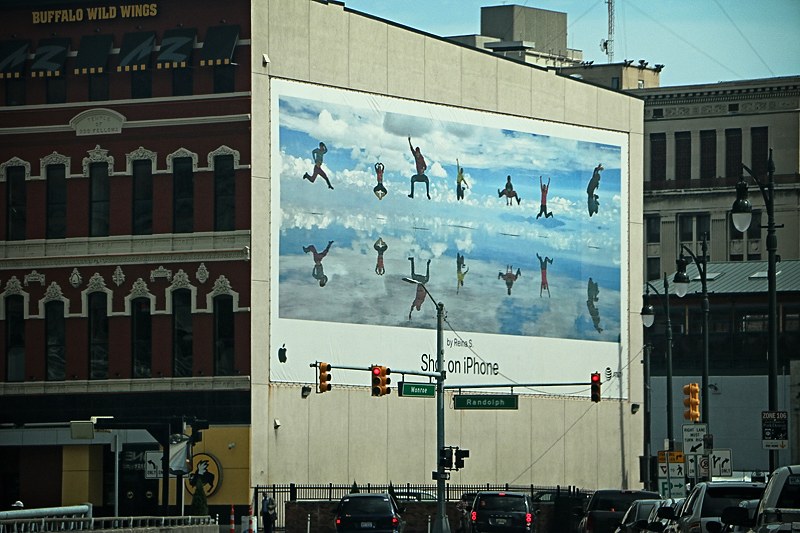This is a vibrant color photograph depicting a striking billboard affixed to the side of a white building. The billboard features a stunning image of a bright blue sky dotted with fluffy white clouds, and showcases two rows of people, each row comprising seven individuals. Overlaying the image, the text reads "Shot on iPhone by Rina S." in bold black letters. In the foreground, a traffic light with attached street signs marks the intersection of Randolph and Western. Both traffic signs are green with white lettering, and the traffic light is currently displaying a red signal. The edifice below the billboard is constructed from red brick with elegant white detailing, adding a classic touch to the urban streetscape. A clear blue sky serves as a serene backdrop to the entire scene.